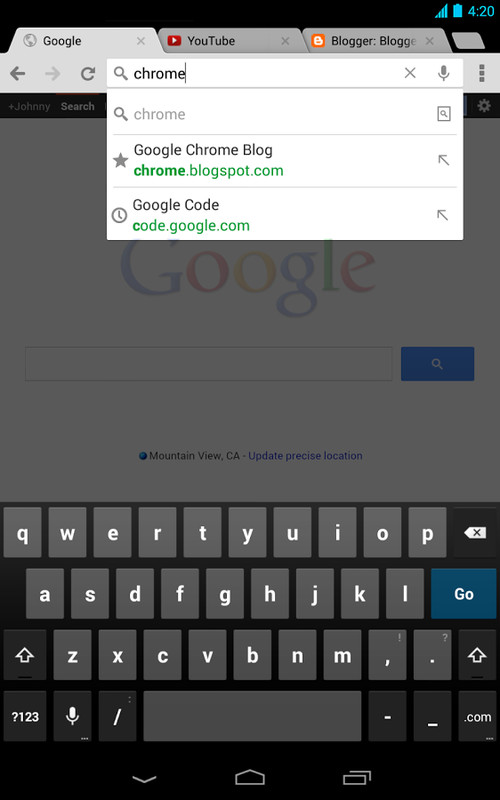The image depicts an Android browser with three tabs open at the top: the first tab is titled "Google," the second "YouTube," and the third "Blogger," which cuts off after "B-L-O-G-G-E." In the top left corner, the device displays several notifications in aquamarine: signal bars, a full battery icon, and the time, "4:20." 

The search bar shows someone typing "Chrome," with the cursor positioned immediately after the last "e." Below the search bar, three search results are visible. The first result, which features a gray magnifying glass icon, simply reads "Chrome." The second result, marked with a gray star, displays "Google Chrome Blog" in black, followed by "chrome.blogspot.com" in green with the word "Chrome" in bold. An arrow points to the upper left beside this result. The third result includes a clock icon and reads "Google Code" in black, with "code.google.com" in green, highlighting a bolded "C." This result also features an arrow pointing to the upper left.

In the background, a faintly visible, traditional Google logo from the early 2000s is set against a white rectangular search area. This vintage logo is sharper compared to its more modern, rounded counterpart. The search area includes a smaller blue rectangle on the right, containing a magnifying glass icon for submitting searches.

At the bottom of the image, an old-fashioned Android keyboard is partially visible. The QWERTY keys have a light gray background, the "Go" button is navy blue, and the remaining keys are dark gray. This keyboard design also appears to be from the early 2000s.